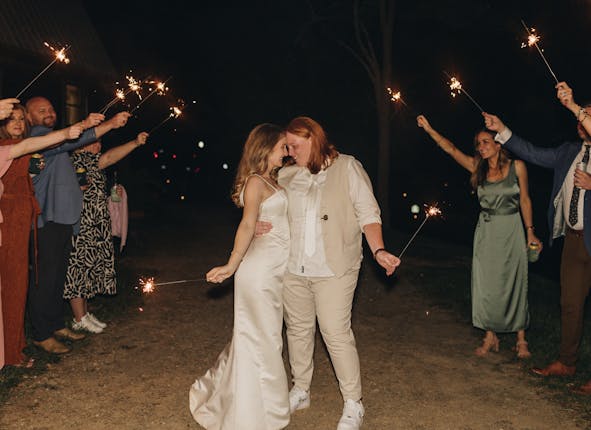In this nighttime outdoor wedding scene, a joyous lesbian couple stands at the center, surrounded by guests holding sparklers that illuminate the celebration. The bride on the left is wearing a traditional satin wedding gown with spaghetti straps and has long brown hair cascading over her shoulders. She stands forehead to forehead with her partner, who is dressed in a cream-colored ensemble consisting of a vest, rolled-up white button-down shirt, satin tie, and pants. The second bride, with her shoulder-length red hair, is slightly chubbier. Both women are holding sparklers, creating a whimsical, glowing atmosphere. Their guests, dressed in a mix of casual and semi-formal attire, form an arch of light with their sparklers, drawing attention to the loving couple at the center. One guest stands out, wearing a suit with a blue jacket and brown pants. The entire scene captures a moment of pure celebration and love under the night sky.